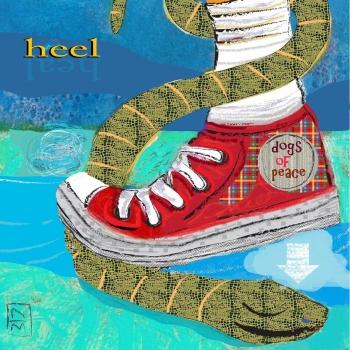The brightly colored, stylized illustration, which bears a resemblance to a children’s book cover, features a dominant blue-green background with various shades swirling in layers. At the forefront, a prominent red high-top tennis shoe with white plastic toe caps and white laces is depicted. The shoe's side panel is adorned with plaid material and an emblem reading "Dogs of Peace." A white sock-covered foot wearing this shoe is being encircled by a greenish snake with small stripes. The snake coils around the foot and extends beneath it, its head positioned just under the shoe's heel. Directly under the heel, a blue cloud with a white arrow indicates the heel is poised to crush the snake's head. In the upper left-hand corner, the word "heel" is printed in small but significant yellow font. The scene has an ethereal quality, possibly underwater, with the color transitioning through different shades of blue and a river-like formation weaving through the composition.